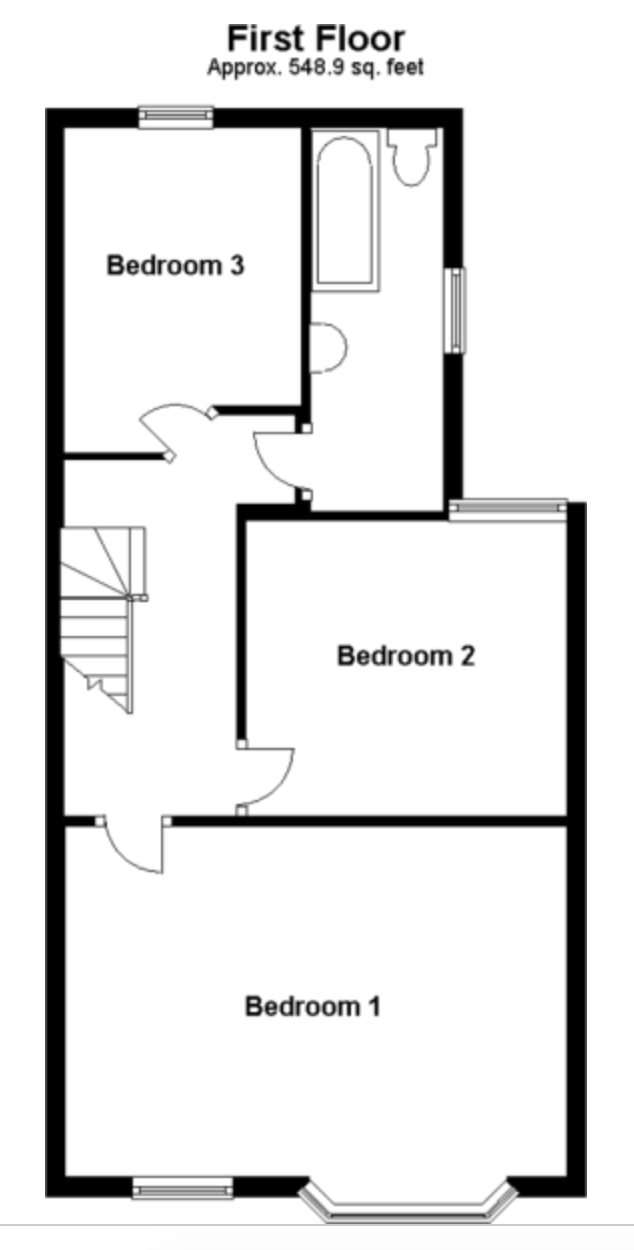This is a detailed sketch of a first-floor apartment featuring a floor plan that spans approximately 548.9 square feet. It includes three bedrooms and one bathroom. The largest bedroom, Bedroom 1, is located at the bottom of the plan and features a door that swings inward. Moving from Bedroom 1, there is Bedroom 2, also accessed via an inward-swinging door. Adjacent to Bedroom 2, there appears to be a small room or possibly attic stairs. This area leads to a hallway connecting to Bedroom 3, which is accessible through another inward-swinging door. 

The bathroom is conveniently situated next to both Bedroom 2 and Bedroom 3. The bathroom layout includes a bathtub and a toilet. Notably, the floor plan does not indicate the location of the kitchen, closets, or any additional storage spaces, and raises questions regarding their placement within the apartment. The entire layout is representative of a compact yet functional living space.